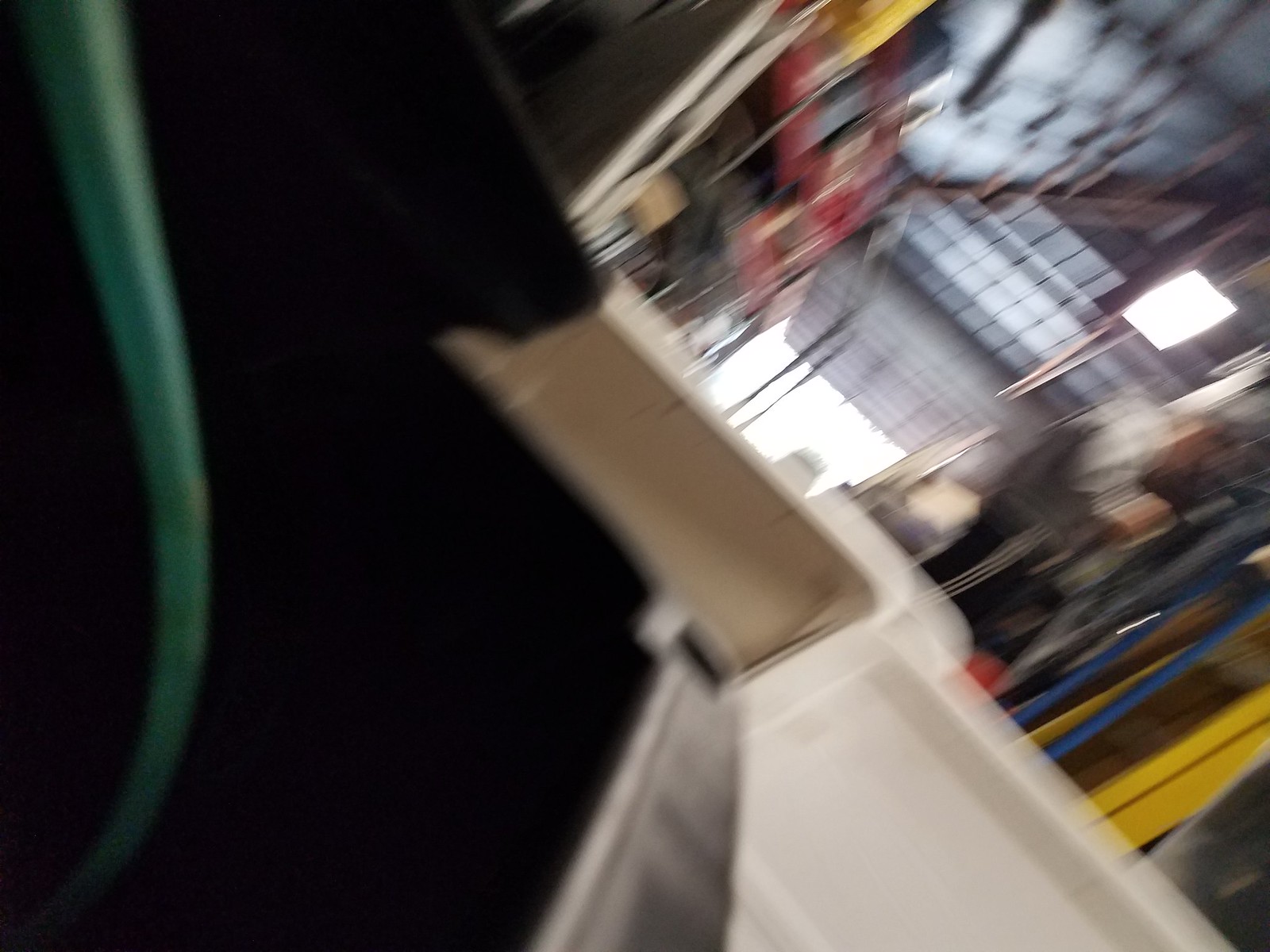The image depicts an extremely blurry interior of what might be a building, possibly a warehouse or a garage. On the left side, there's a vertically oriented green cylindrical shape, likely an extension cord, extending from the top to the bottom of the frame. Adjacent to this is a dark, black region occupying about a third of the image’s left side. A white-colored shape appears to connect to this black area, resembling a paneled wall or possibly part of a truck bed. The roof of the structure is visible, showcasing unfinished beams and potentially a skylight.

The surrounding environment is very colorful, with various blurred objects in hues of yellow, blue, and red scattered throughout the scene. These colors might belong to stacked items or tall shelving units common in large storage facilities like a Costco. The right side features vertical objects in blue and yellow, while the left side includes red, square-shaped items positioned higher up. The center of the image is brightly lit with a noticeable white light, and there seems to be an open space that leads to the outdoors, potentially with a vehicle visible outside. The overall brightness and unclear details make it difficult to precisely identify all elements, with some areas displaying a checker-like pattern that adds to the complexity.